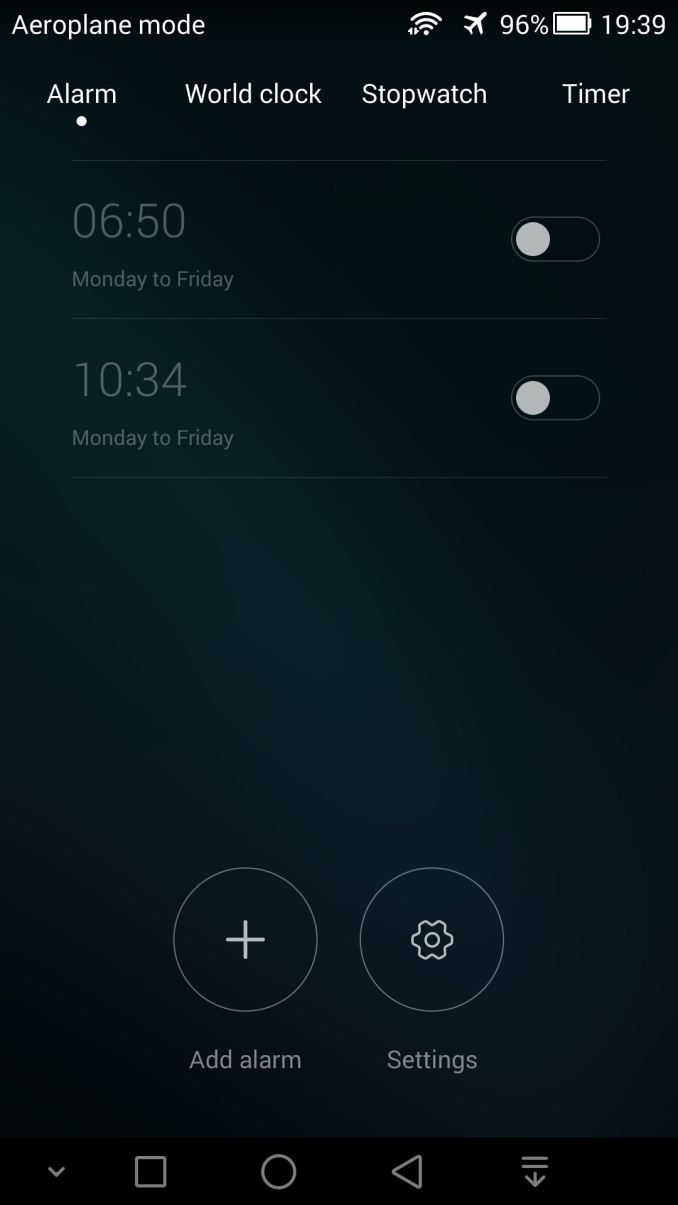This is a detailed screenshot of a mobile phone's settings interface. At the top of the screen, "Airplane Mode" is displayed with a corresponding airplane icon on the right side. The battery level is shown at 96%, and the current time is 19:39. Below is a navigation menu featuring options for Alarm, World Clock, Stopwatch, and Timer, with the Alarm option presently selected, indicated by a white dot beneath it.

Under the Alarm section, two alarms are listed: one set for 06:50 and the other for 10:34, both scheduled to go off Monday through Friday. The screen has a black background with white text, while the alarm times are depicted in gray. Further down, there's a circle containing a plus sign, labeled "Add Alarm," adjacent to another circle with a gear icon labeled "Settings."

At the very bottom of the screen are the standard navigation icons of a mobile phone: a square for recent apps, a circle for the home screen, and an arrow pointing left for back.